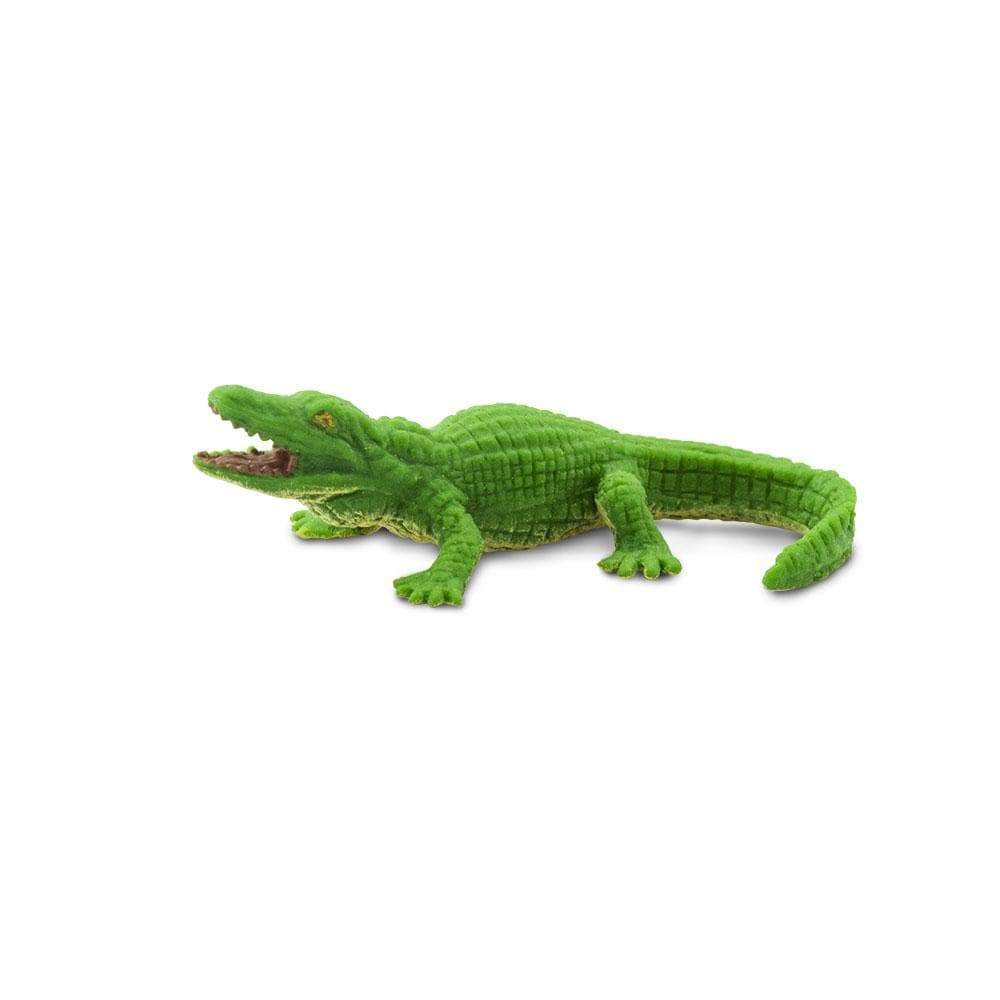The product photograph, intended for commercial use, features a toy alligator placed against a stark white background and surface, ensuring the focus remains solely on the product. The alligator, positioned in profile and facing left, is crafted in a stylized design. Its body is predominantly neon green, resembling lime green, with a yellow underbelly and eyes. The scales are intricately carved into square patterns, adding to the toy's textured appearance.

The alligator is depicted with an open mouth, showcasing white, zigzag-shaped teeth and a pink interior. Its four legs, with five toes each, are splayed out, simulating a walking motion. Notably, the toy's tail curves towards the right side of the image, with a slight portion extending beyond the frame. The alligator’s overall appearance and detailing, including the unrealistic eyes and rubber-like texture, suggest it is a children’s toy designed more for play than realistic representation. The image composition adheres to a Photographic Representationalism Realism style, presenting the toy with a lifelike clarity despite its distinctly playful and imaginative design.